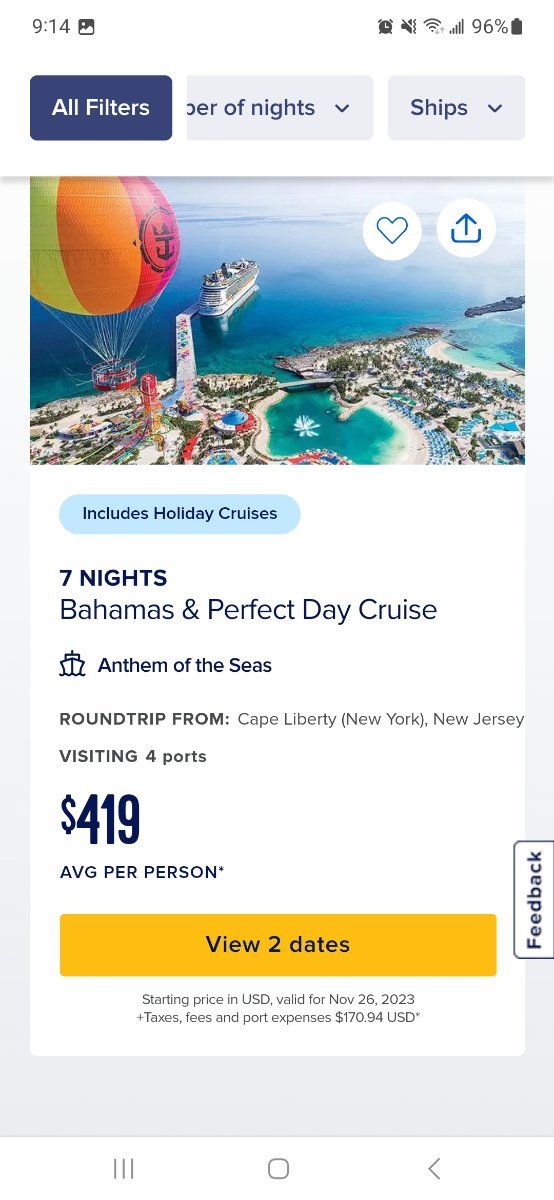This is a screenshot from a travel app, featuring the phone's UI at the top, displaying the time on the left, an image icon, and a battery life indicator at 96%. Below this, there are three filter options: a dark blue "All Filters" box, a partially visible "Number of Nights" dropdown, and a "Ships" dropdown. The main image below these options is an aerial view of a tropical beach with white sand and crystal-clear water. A hot-air balloon floats over the beach, and a cruise ship is departing from the shore. Below the image, there's a light blue, pill-shaped button that reads, "Includes holiday cruises." Under this button, another text reads, "Seven Nights Bahamas and Perfect Day Cruise."